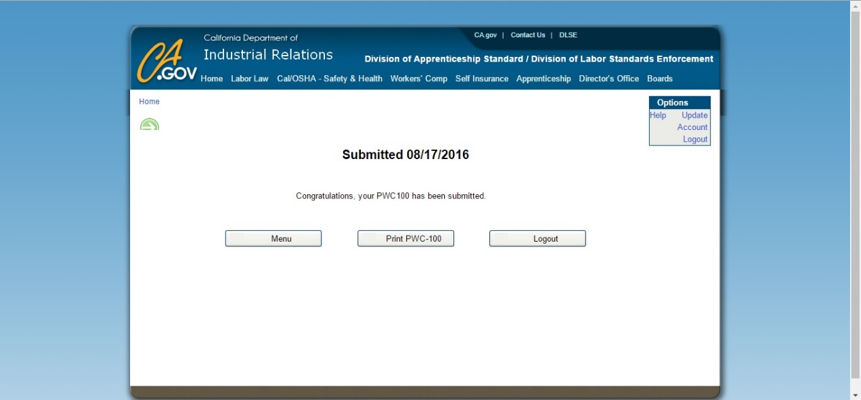The image features a webpage with a light blue background and a prominent dark blue header at the top. The header contains the official branding for CA.gov, along with the text "California Department of Industrial Relations." There are also clickable links for "CA.gov," "Contact Us," and "DLSE" (Division of Labor Standards Enforcement). 

Directly below the header, the webpage displays the title "Department of Apprenticeship Standards / Division of Labor Standards Enforcement." Following this title, there is a navigation menu with options including Home, Labor Law, Cal/OSHA, Safety and Health, Workers' Comp, Self Insurance, Apprenticeship, Director's Office, and Boards.

The main content area of the page is set against a white background. At the top of this section, it reiterates the "Home" link. Below, there is a contextual box containing options like Options, Help, Update Account, and Logout.

Centrally placed on the page is text indicating the submission date: "Submitted 08/17/2016." A few lines further down, it congratulates the user with the message: "Congratulations, your PwC 100 has been submitted." There is also a navigation box labeled "Menu" and two additional buttons - one for printing the PwC-100 form titled "Print PwC-100," and another for logging out, labeled "Logout."